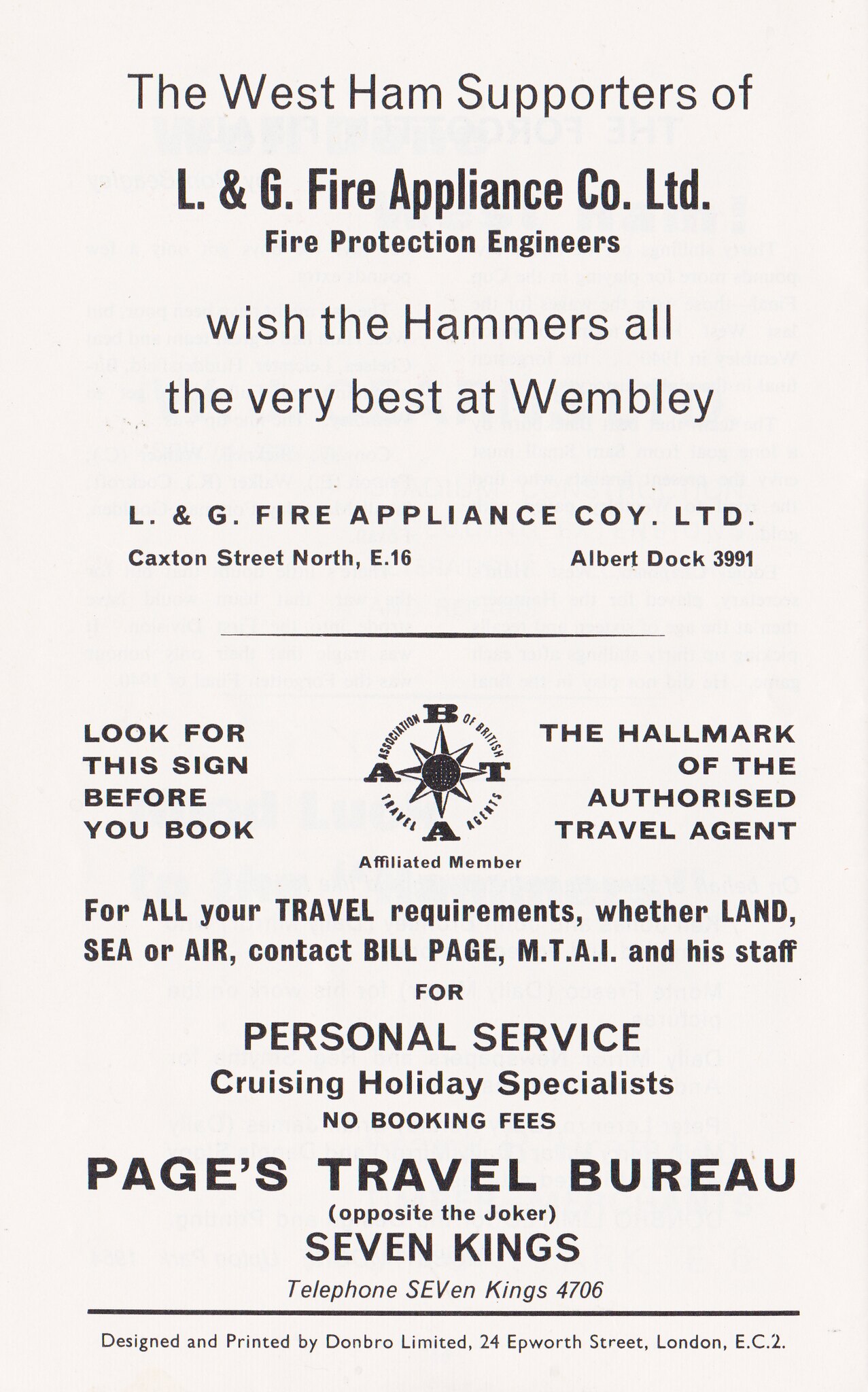This image features an off-white-pink or cream-colored flyer with black text. At the top, it reads, "The West Ham supporters of L&G Fire Appliance Company Limited Fire Protection Engineers wish the Hammers all the very best at Wembley." This message is from L&G Fire Appliance Coy Ltd, located at Caxton St North E16, Albert Dock 3991. Below, a horizontal black line divides the flyer.

On the left side, it says, "Look for this sign before you book." In the center, there is a logo resembling a compass rose or eight-pointed star with the initials "A, B, T, A" at the cardinal points, representing the Association of British Travel Agents. This is described as "the hallmark of the authorized travel agent."

Below, for all your travel needs by land, sea, or air, you are encouraged to contact Bill Page, MTAI, and his staff at Page's Travel Bureau for personal service, specializing in cruising holidays with no booking fees. The bureau is located opposite the Joker in Seven Kings, with a telephone number listed as 7 Kings 4706. The flyer mentions being designed and printed by Dombro Limited, London.